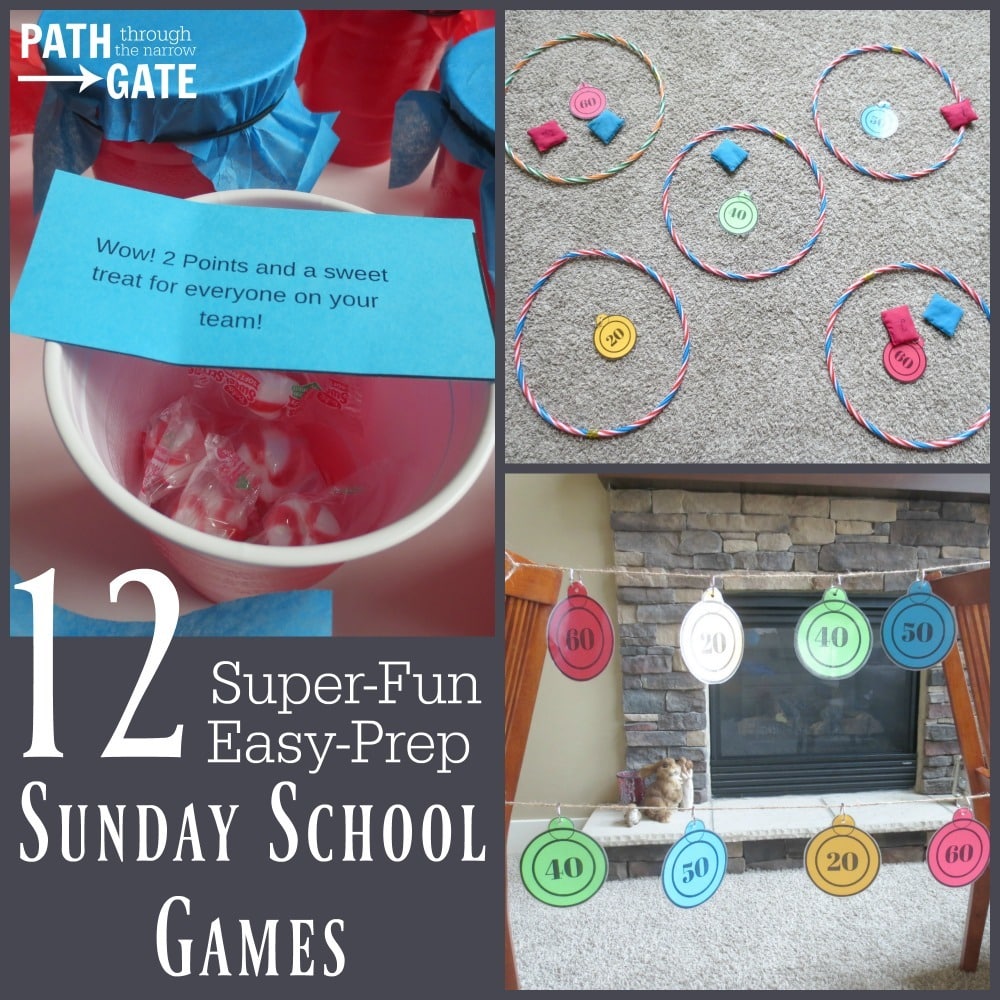The image is a poster divided into four sections featuring information and visuals about 12 super fun, easy prep Sunday school games. The text on the top reads "Pathgate through the narrow" in white letters on a gray background, while the bottom features a larger white caption, "12 super fun, easy prep Sunday school games." On the upper left of the poster, there is an image of a plastic cup, resembling a Dixie cup, with a piece of paper on top that reads, "Wow, two points and a sweet treat for everyone on your team."

In the upper right section, the image depicts a gray carpet where circular wire hoops lie, each containing round tokens labeled with point values of 10, 20, and 60. Red and blue beanbags are scattered around, indicating that participants likely throw the beanbags into the hoops to score respective points. 

Below this, there is another image showing chairs with strings strung between them, and round targets hanging on the strings, similar in appearance to the tokens in the upper right. These targets have varying point values and appear to be positioned for a game where attendees aim to hit the highest point target. The background of this lower image features a fireplace, adding a cozy, indoor setting to the described games.